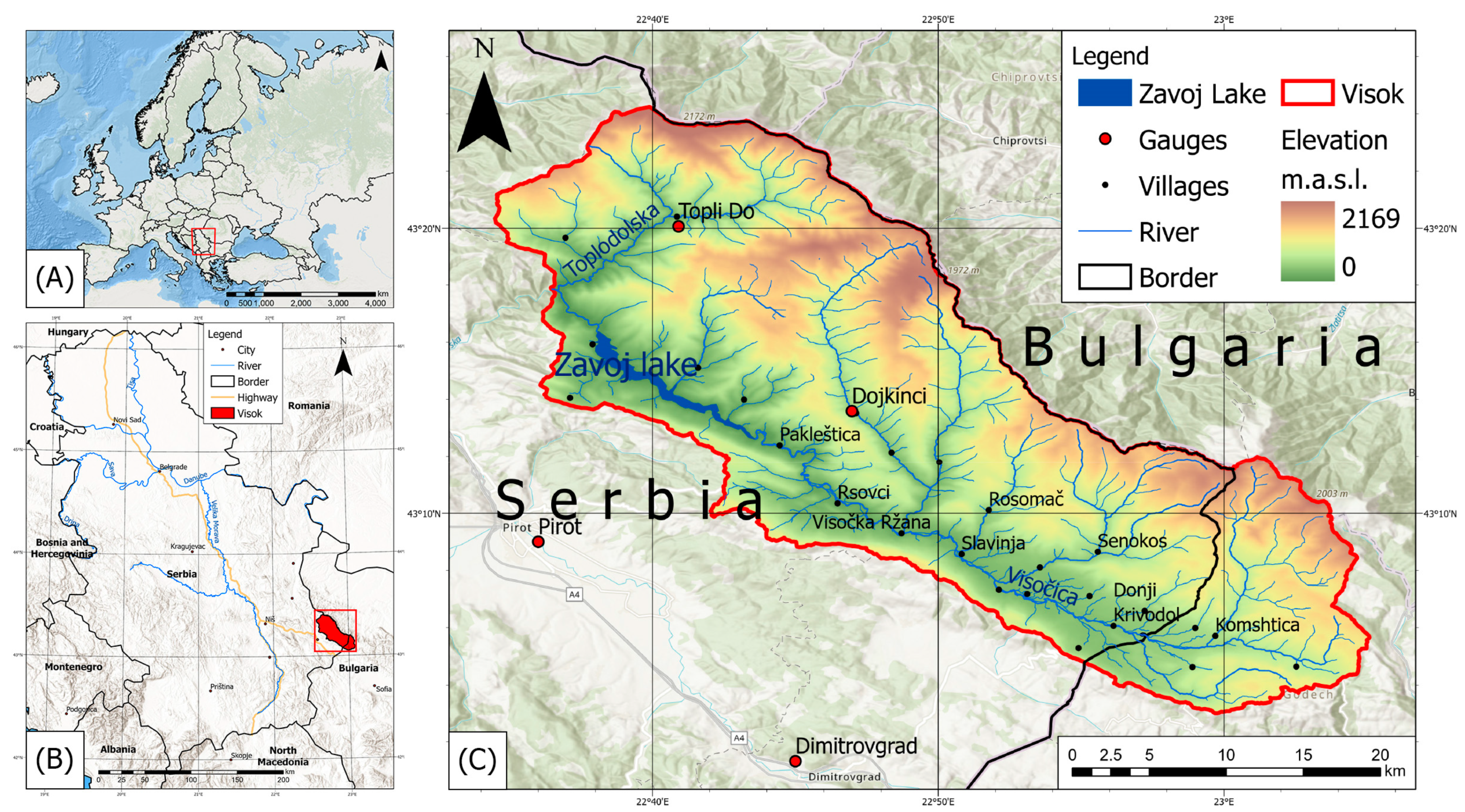The image consists of three maps labeled A, B, and C, each serving a different purpose in detailing a geographic region. 

**Map A**, located in the top left corner, is a broad map of Europe featuring a faintly colored, gray and blue depiction. A red square prominently marks an area in the southern part of Europe, specifically around Serbia and Bulgaria.

**Map B**, positioned directly below Map A, focuses on the finer details of the highlighted region and includes a legend. It displays a grayscale map with black lines indicating borders and various geographic features. According to the legend, blue lines represent rivers, black rectangles symbolize borders, orange or yellow lines signify highways, and red rectangles denote particular areas of interest such as Vistach.

**Map C**, the most detailed and largest map on the right, zooms in on the region between Serbia and Bulgaria. It features a multicolored, rainbow-like elevation heat map outlining the terrain in detail. The map uses a spectrum of colors from blue to green, orange, and yellow to illustrate different elevations, with areas outlined in red signifying the specific focus area between the two countries.

Overall, the image effectively narrows from a broad view of Europe to a detailed geographic analysis of a specific region between Serbia and Bulgaria, highlighting topographical and infrastructural elements.